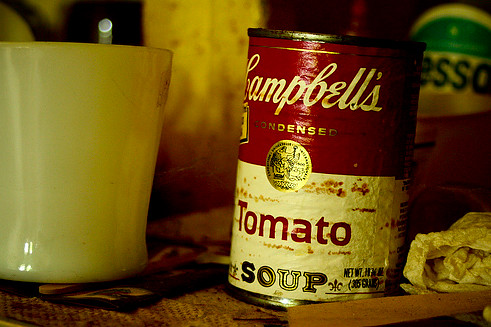A close-up view showcases a weathered and distressed can of Campbell's Tomato Soup, with noticeable rust marks on the can and its label. The top of the label features "Campbell's" in iconic scroll letters, while the white section below reads "Tomato Soup" with "Tomato" in red letters and "Soup" in gold. A central crest separates the red upper half of the can from the white lower half. Though the net weight is partially obscured, it reads "300 and something grams" in black text. The can's label appears crinkly, indicative of age and possible water damage.

To the right of the can is a vintage-looking white coffee mug resting on an aged piece of fabric. In the background, an old jar of Wesson Cooking Oil, with a vintage green and white label, can be seen. The foreground is cluttered with pieces of fabric and bits of wood, adding to the rustic, nostalgic atmosphere of the scene.